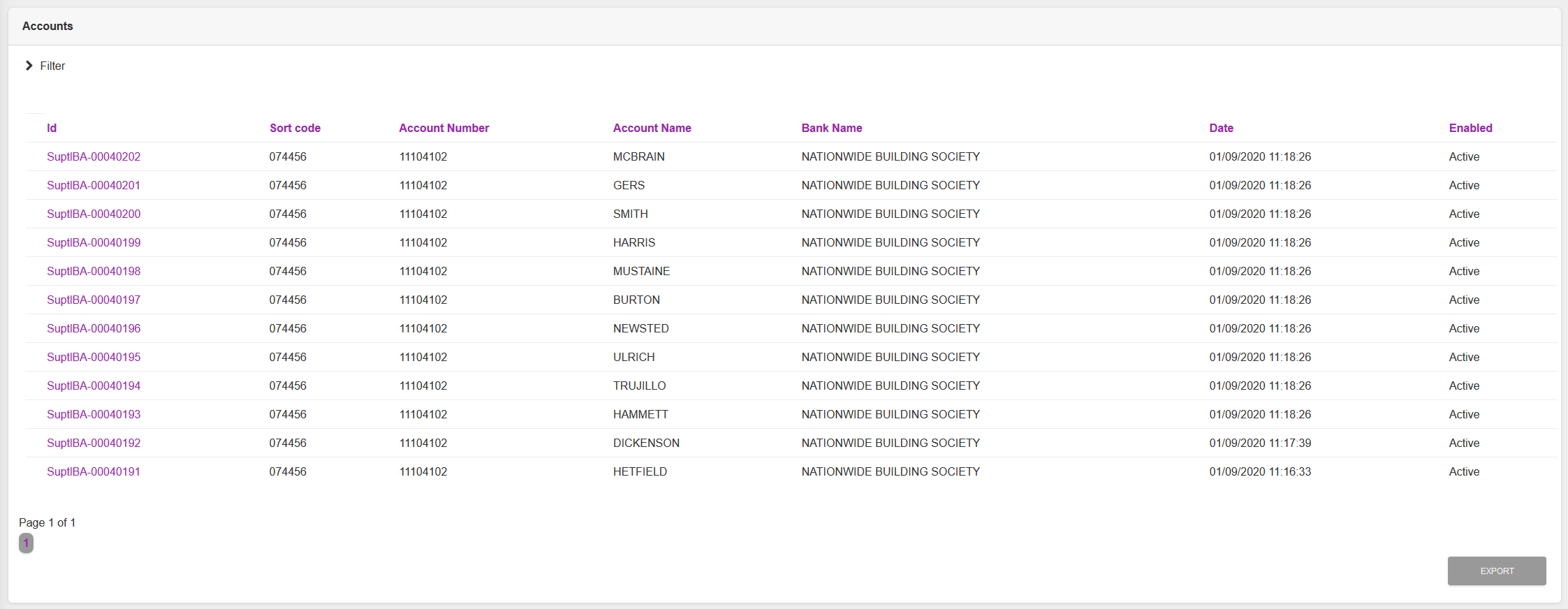This image is a screenshot from a website displaying a document-like interface with a clean, white background. In the upper left-hand corner, there is a label that reads "Accounts," and just below it, an option for "Filter." The interface is organized into various columns, starting with "ID," which lists different identification numbers in purple text. The subsequent columns are "Sort Code" and "Account Number," both of which repeat the same numbers across different IDs. Further along, there is an "Account Name" column, where all the column headers are in purple text and the entries are in black.

Notably, the "Account Name" column features names of individuals associated with heavy metal bands, particularly Iron Maiden and Metallica. Examples include "McBrain" (referring to Nicko McBrain, drummer for Iron Maiden), "Gers" (Yannick Gers, Iron Maiden guitarist), and "Harris" (Steve Harris, Iron Maiden bassist). Additional names from Metallica's lineup also appear, such as "Mustaine" (Dave Mustaine), "Burton" (Cliff Burton), "Ulrich" (Lars Ulrich), and "Trujillo" (Robert Trujillo).

The page header also includes a bank name, "Nationwide Building Society." Another column, "Date," and an "Enabled" status indicator follow the account names. 

In the bottom right-hand corner, there is a gray button with the word "Export" in white text. All data entries are meticulously organized, creating a structured and informative display.